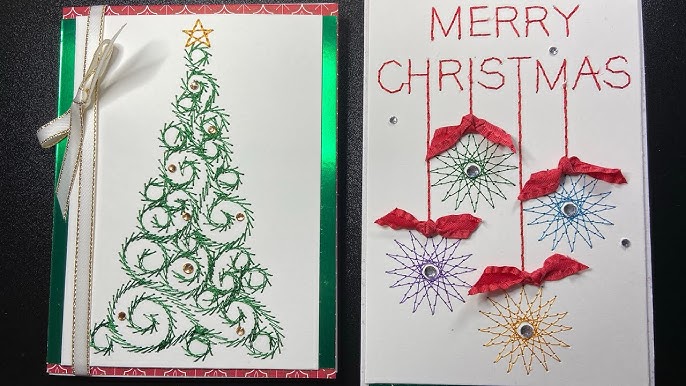In the photograph, two vibrant handmade Christmas cards are set against a flat black background, exuding festive cheer with their intricate designs. The card on the left showcases a unique, raised, swirling Christmas tree made of dark green wire or thread, adorned with bronze sequins or beads, and crowned by a gold star. This card also features a vertically positioned white ribbon with gold trim running along its folded edge. The card on the right, equally colorful, prominently displays the words "Merry Christmas" crafted from thread. From the letters H, I, T, and M, red ribbons cascade down to intricate, multi-pointed stars, each centered with a diamond-like gem. Both cards are meticulous in design, capturing the essence of handmade artistry.